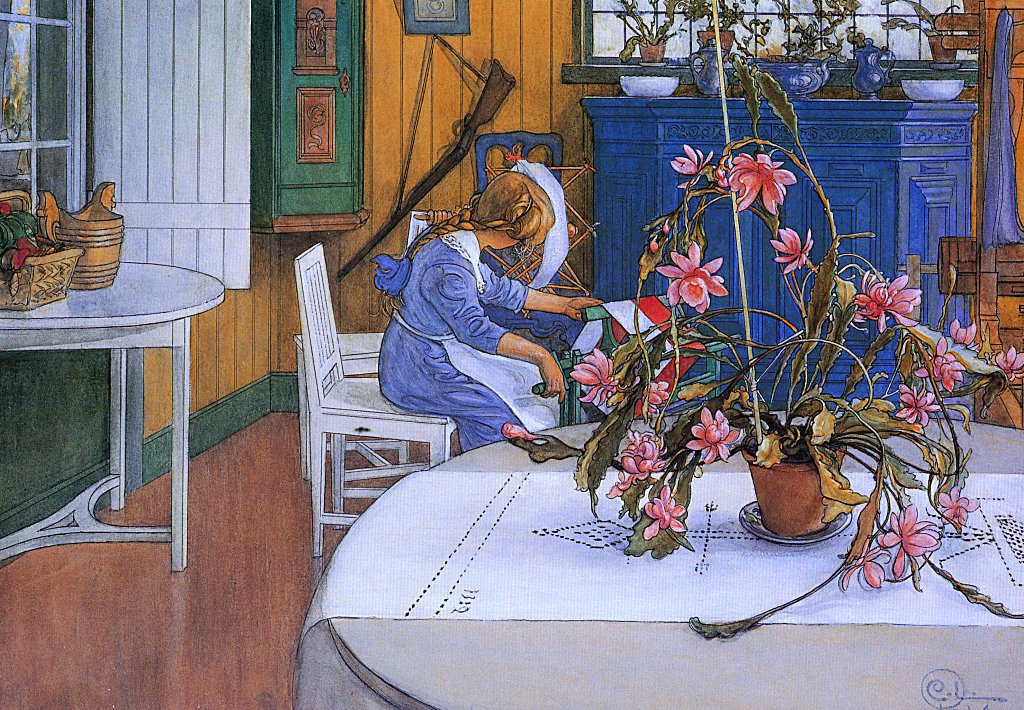This detailed watercolor painting from 1914, titled "Interior with a Cactus," portrays an old-fashioned, rustic living or dining room setting in meticulous detail. The focal point is a young girl with a long, amber-colored braid tied in a blue ribbon, sitting on a white chair. She is dressed in a blue dress with a white apron and is engrossed in some type of handicraft, possibly operating a loom or a similar piece of equipment with red and white material. Her face is turned away from the viewer, giving a view of the back and the right side of her face.

In the foreground, there is a circular table with a white runner and brown lettering, centered with a small brown pot containing a large flowering cactus with pink roses. Some leaves appear to be turning brown and dying, supported by a rod. The floor below is a reflective brown, and the base of the wall has a green trim.

Behind the girl, to the left, there's another round table with white legs, topped with a wooden and a square wooden bowl. This table is placed in front of a window with open wooden blinds. Further to the right, there is a dark blue china cupboard with white bowls on the sides and green bowls in the center. Above it, through the window, several flower pots are visible.

The setting also includes a wooden paneled wall with a 19th-century vintage rifle hanging from a nail, and above it, a blue picture frame. To the right, there’s a teal-colored cabinet. The household’s tidy and clean aesthetic is evident throughout this piece. In the bottom right corner, there's a signature in blue freehand, starting with a C encircled by a loop, though the rest is illegible.

This painting beautifully captures a serene, rustic interior from a bygone era, emphasizing simplicity and the charm of early 20th-century farmhouse life.